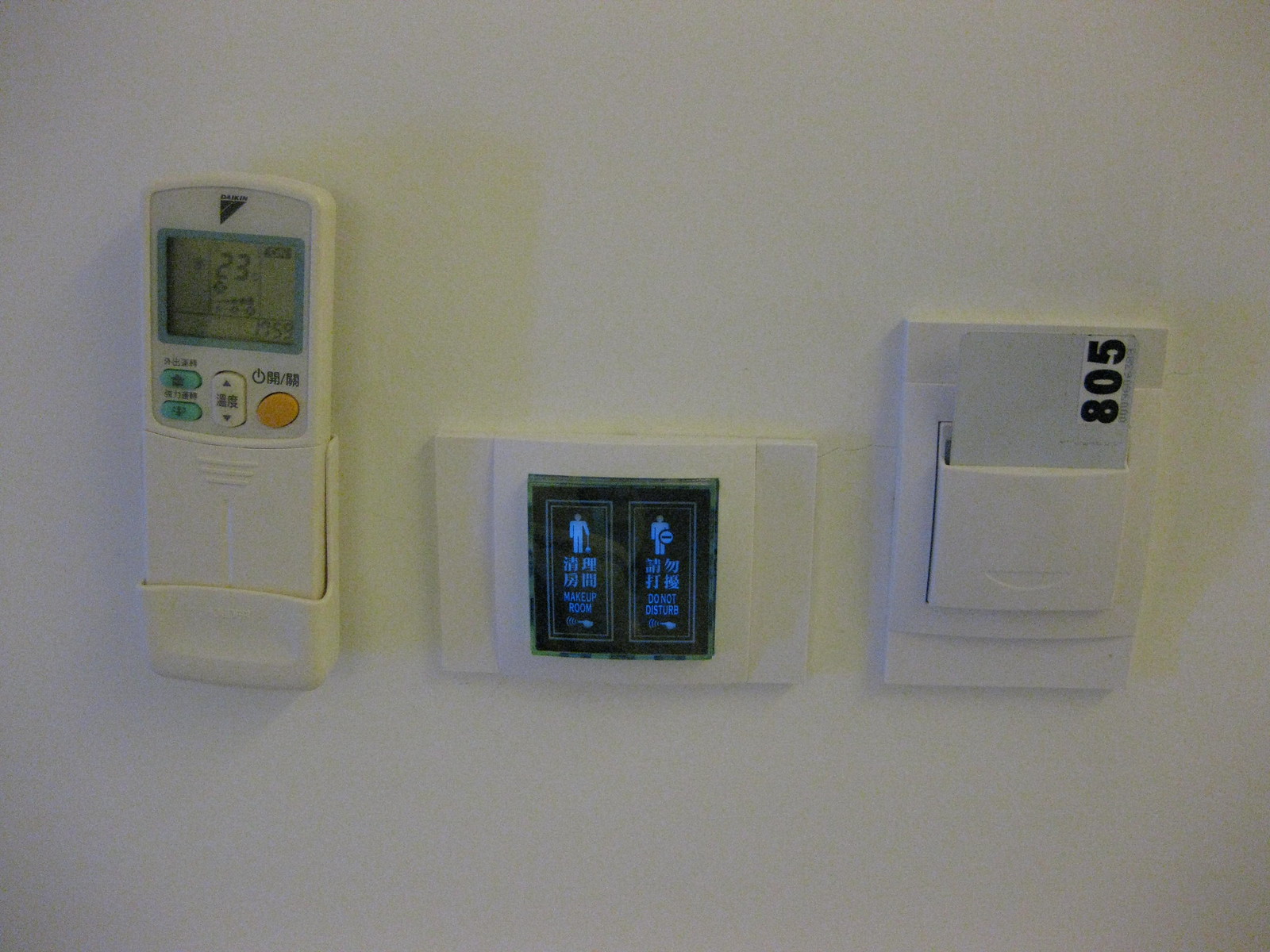The image depicts a wall with three mounted items arranged from left to right. 

On the left side, there is a holder designed for an air conditioning and heating unit remote. Both the holder and the remote are off-white in color. The front of the remote features a ridged section, likely a battery compartment cover, which can be slid downwards. Above this section, two blue buttons are positioned on the left; one button is marked with a snowflake, suggesting a cooling function, while the other has a different symbol, possibly representing heating. The center of the remote has a button with up and down black triangles for temperature adjustment, and on the right side, there is a yellowish button with a black power symbol for turning the unit on or off. The top of the remote has a small greenish display screen bordered with a grayish-blue rim, showing black text. Above the screen, a partially visible black logo, somewhat triangular in shape, is present, though the text above it is difficult to read.

In the center of the image, a white panel is mounted on the wall. It has a central black square screen with two sections. The left section displays a symbol of a person holding a broom, with the label "Makeup Room" and an arrow pointing to the right beneath it. The right section features a symbol of a person with a prohibition circle (a circle with a line through it) where the broom symbol was, labeled "Do Not Disturb."

On the right side, another wall-mounted holder contains a piece of paper. The visible top-right (bottom-left when facing it) corner of the paper displays the number "805."